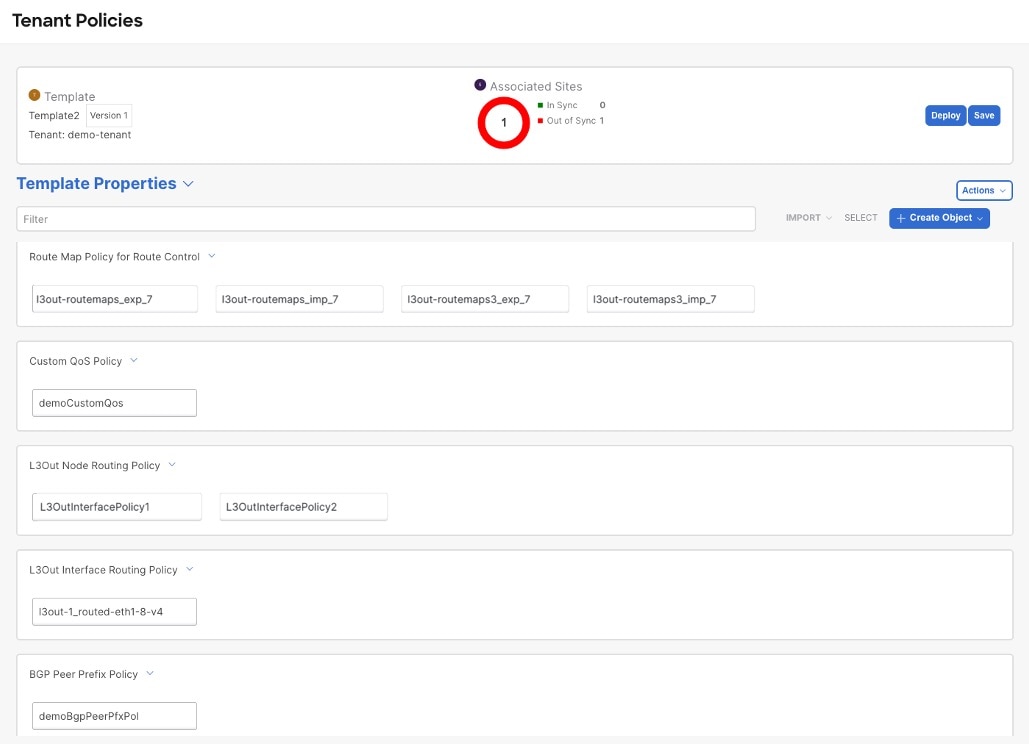The image displays a detailed interface for managing tenant policies. On the left side of the screen, there's a menu with the heading "Tenant Policies." Below this heading, "Template" is listed, followed by entries "Template 2 Version 1" and "Template Demo Tenant."

In the middle of the screen, there are sections detailing the synchronization status of associated sites. It shows “Associate Sites: In Sync 0, Out of Sync 1” with a red circle indicating the out-of-sync status.

Below this, there are options for "Display and Save." The "Template Property" section features a filter option, followed by the listing "13 Out Route Maps EXP_7" repeated four times.

Below these listings, there's a drop-down arrow next to "Custom OOS Policy," followed by "Demo Custom OOS." Further down, another drop-down arrow is shown next to "L3DUT Node Routing Policy," under which "L3OUT Interface Policy 1" and "L3OUT Interface Policy 2" are listed. There is another drop-down arrow for the "L3OUT Interface Routing Policy" section, and finally, the "BGP Fever Prefix Policy" is mentioned.